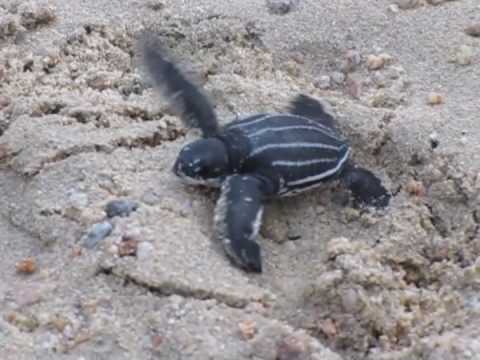In the photograph, a small sea turtle is captured making its way across the sandy bottom of a marine environment. The turtle is predominantly black with striking white stripes decorating its shell, which is shaped somewhat like a sunflower seed. Its head is entirely black, and its flippers, bordered in white, suggest it's used to swimming, although it currently appears to be crawling.

The substrate under the turtle is composed of light brown, fine sand that looks characteristic of a beach setting. Scattered across the sandy expanse are numerous seashells and pebbles: notable mentions include blue, white and blue, and brown shells, as well as multicolored shells in the upper left corner. Some areas of the sand display a hilly texture with more cracks and agitation, especially near the top left and bottom right of the image.

Interestingly, there is a fine black smoke-like substance visible emanating from beneath the turtle’s left front fin, rising towards the left center of the image. This could hint at a defensive action or some interaction with the sand and water around it. The turtle's motion is directed from the bottom right corner towards the bottom left, its flippers poised as though it's propelling itself in an aquatic environment.